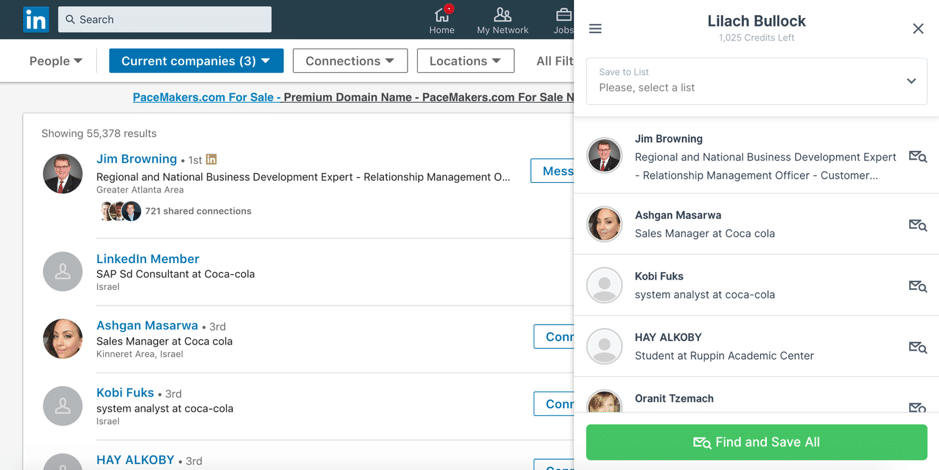The image is a split screen showing an Indeed search page on the left and a user profile on the right.

On the left side:
- The Indeed logo is positioned at the top left corner followed by a search bar. The "Current Companies" tab is highlighted.
- Below the search bar, search results are displayed:
  1. The first result features a photo of a middle-aged businessman within a circle, identified as Jim Browning. His details include: "Regional and National Business Development Expert, Relationship Management, Greater Atlanta Area, 721 Shared Connections."
  2. The second result shows a circle with a generic person icon and the description: "LinkedIn Member, SAP SD Consultant at Coca-Cola, Israel."
  3. The third result displays a woman's icon with the name "Ashken Masarwa, Sales Manager at Coca-Cola, Kinneret Area, Israel."
  4. The fourth result is another circle with a generic person icon, labeled: "Kobe Fuchs, System Analyst at Coca-Cola, Israel."

On the right side, the user profile:
- The profile belongs to Lilac Bullock, showing "1,025 credits left" at the top.
- There is a dropdown menu labeled "Save to List" with the prompt "please select a list."
- Two photos are displayed below:
  1. Jim Browning, the same businessman from the search results.
  2. Ashken Masarwa, the sales manager from the search results.
- At the bottom, a green rectangle button reads "Find and Save All."